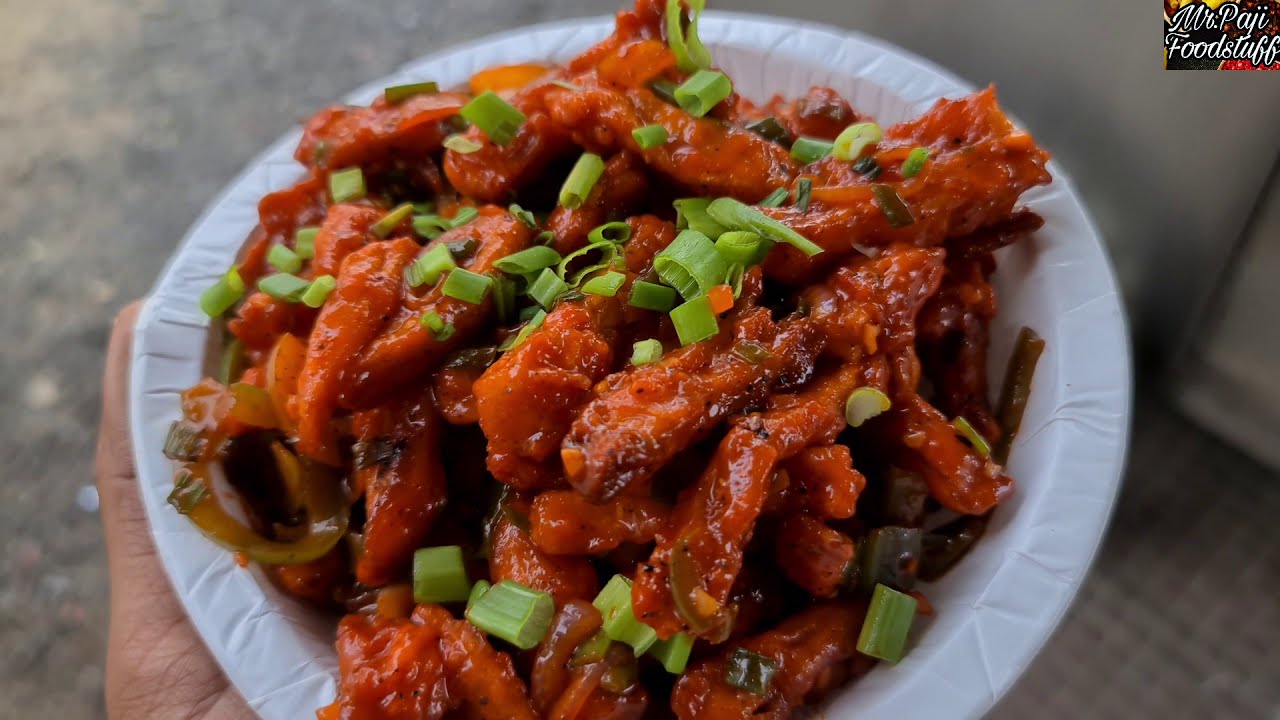The image captures a close-up of a white paper plate filled with a generous portion of what appears to be glazed chicken or possibly pork, covered in a reddish-orange sauce that suggests either a barbecue, hot wing, or Korean spicy flavor. Sprinkled on top of the meat is a dark green garnish, possibly scallions, adding a touch of color to the dish. In the upper right-hand corner of the image, "Mr. Podgy Food Stuff" is written in white, set against a gray background that might be a gravel surface, floor, or even a carpet with a crisscross pattern. The plate is slightly cut off at the bottom, and there's a visible hand holding it on the left side. The gray and brown tones of the background remain blurred, contrasting with the vibrant, detailed food in the forefront.